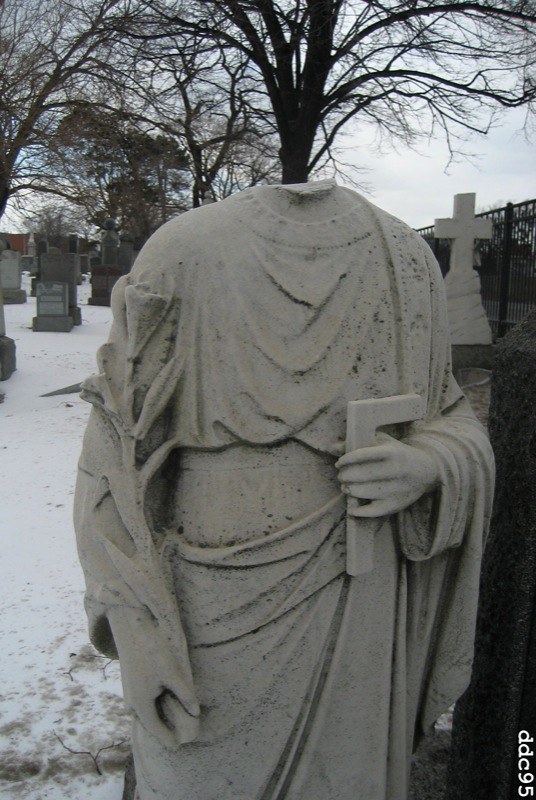This outdoor photograph captures a somber winter scene in a cemetery. The snow-covered ground appears aged and uneven, with patches of darkness disrupting its pristine whiteness. Gray-colored tombstones extend along the left side of the photo, while leafless trees frame the top of the image, their bare branches adding to the stark atmosphere. 

Dominating the central part of the photograph is a stone statue of a saint, rendered in an off-white, gray hue. The statue, however, is damaged—its head is missing, and the figure clutching a long-stemmed flower in its right hand appears forlorn. The left hand of the statue holds what looks like an upside-down L-shaped piece, likely remnants of a broken cross. To the right of the statue, a large tombstone features a prominent white cross, contrasting sharply with the overall muted tones. On the far right, a black metal fence completes this melancholic winter tableau.